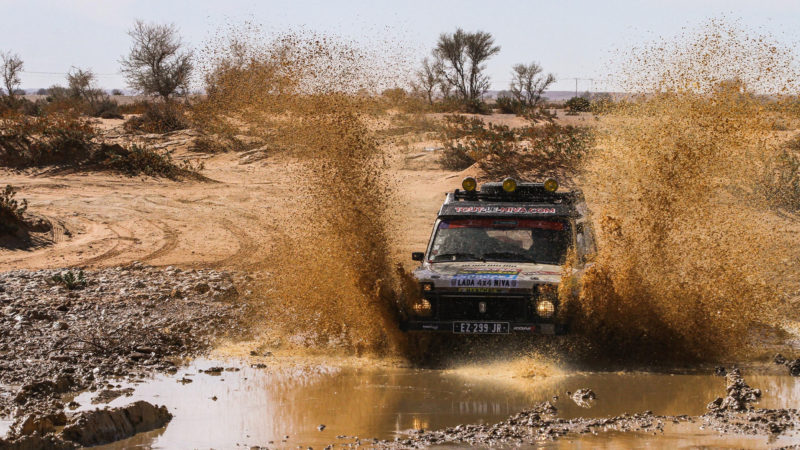A rugged off-road adventure captures a large truck navigating through a muddy, shallow water path, creating an impressive spectacle as brown water and black mud spray up dramatically on both sides. The vehicle, reminiscent of a sturdy jeep or pickup, is adorned with a blue section on the hood displaying "LADA 4x4" in bold black text. A distinctive black license plate reading "EZ299JR" is prominently visible at the front. The truck's hood features three bright yellow lights, adding to its dominant presence, while its headlights shine brightly, illuminating the scene. A red, blue, white, and yellow sticker is affixed above the windshield, colors contrasting amid the rugged terrain. The background of the image reveals a sandy, dirt-laden landscape with sparse vegetation and trees adorned with a sprinkling of leaves. Distant mountains line the horizon under a clear sky with a bluish-gray hue. The overall picture vividly portrays the truck's encounter with the challenging and untamed environment, highlighting the thrill and intensity of off-road driving.